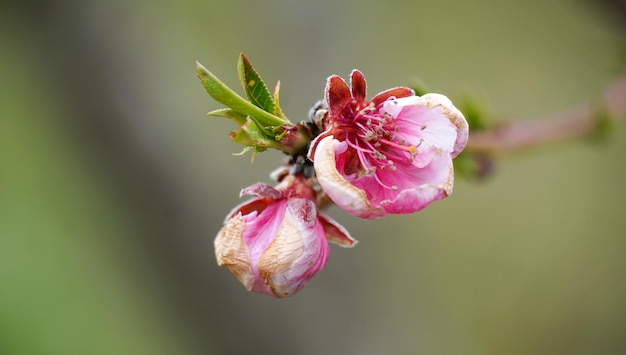This image is a mesmerizing macro photograph focusing on a pink and white flower. The flower in the foreground is fully bloomed, with delicate petals and prominent stamens at its center. Besides this, there is a second flower which remains a bud, facing downward. Between these two flowers, several small, vibrant green leaves emerge, adding a fresh contrast to the scene. The flowers grow from a brown stem that extends into the backdrop, which becomes artfully blurred, creating a professional bokeh effect. The blurred background consists of hues of light green, dark green, and black, likely indicating leaves from the same or nearby plant. The overall composition emphasizes the intricate details and delicate beauty of the flowers and leaves, making for a stunning and intimate nature photograph.